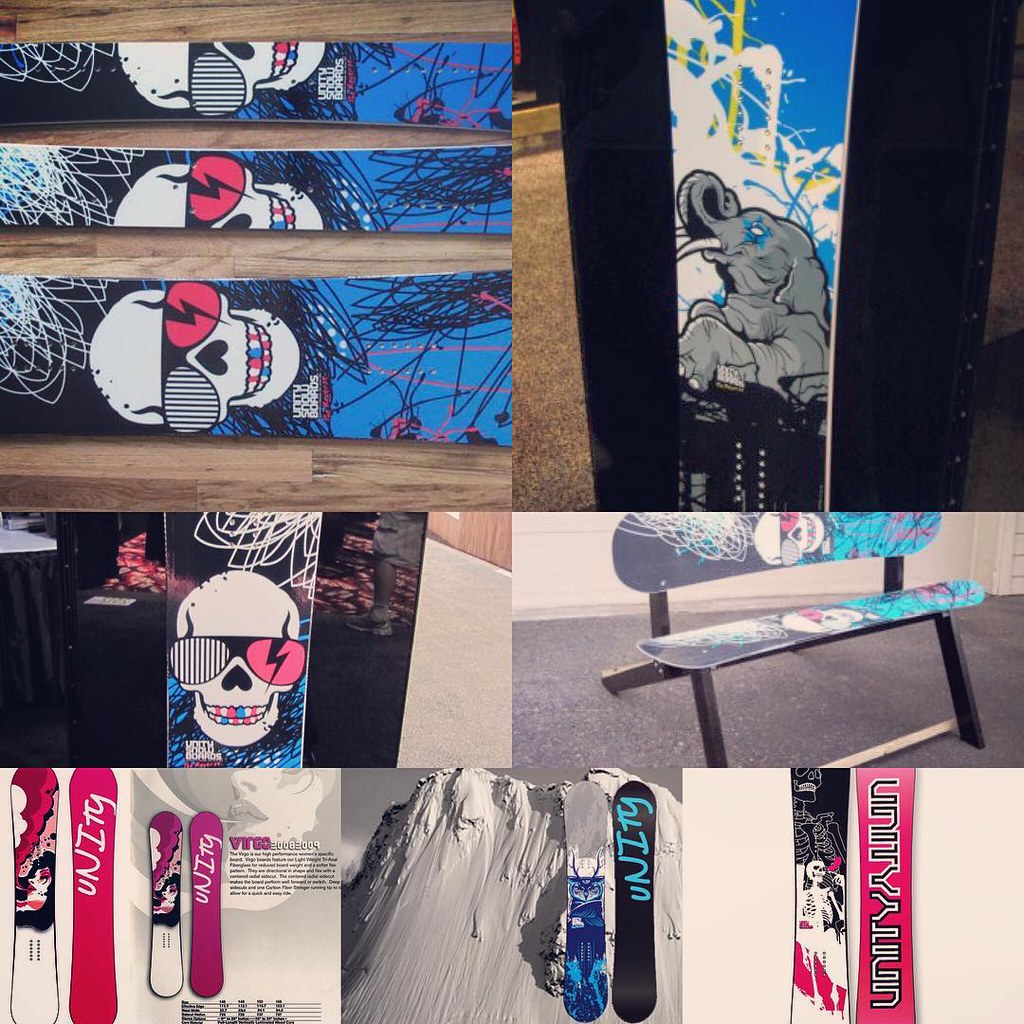The image is a detailed collage of seven photos primarily showcasing snowboards, which share a common branding theme from Unity snowboards. Dominating the visuals, several of the boards feature a distinctive graphic of a white skull with an upside-down heart-shaped nose. The skull's teeth are multi-colored, blending shades of white, pink, red, and blue. The skull wears sunglasses, with one lens sporting black and white stripes and the other a red lens with a lightning bolt. 

The background imagery often looks marker-scratchy with white scribbles or vibrant color fields, adding a raw, artistic touch. One snowboard prominently features an elephant with a blue patch around its eye on a blue background with additional white scribbles. Another notable element is a bench crafted from snowboards, highlighting the skull design and further emphasizing the Unity branding.

In the lower section of the collage, three images present more graphic layouts which seem to serve as advertising for Unity. One image shows snowboards with a red and pink color scheme and a girl's face superimposed over a clouded sky. Another depicts the top and bottom views of a blue and black board against a backdrop of a steep mountain face, and finally, the Unity logo is clearly visible on another board adorned with the skull graphic. Smaller text appears throughout the images but is too minute to decipher.